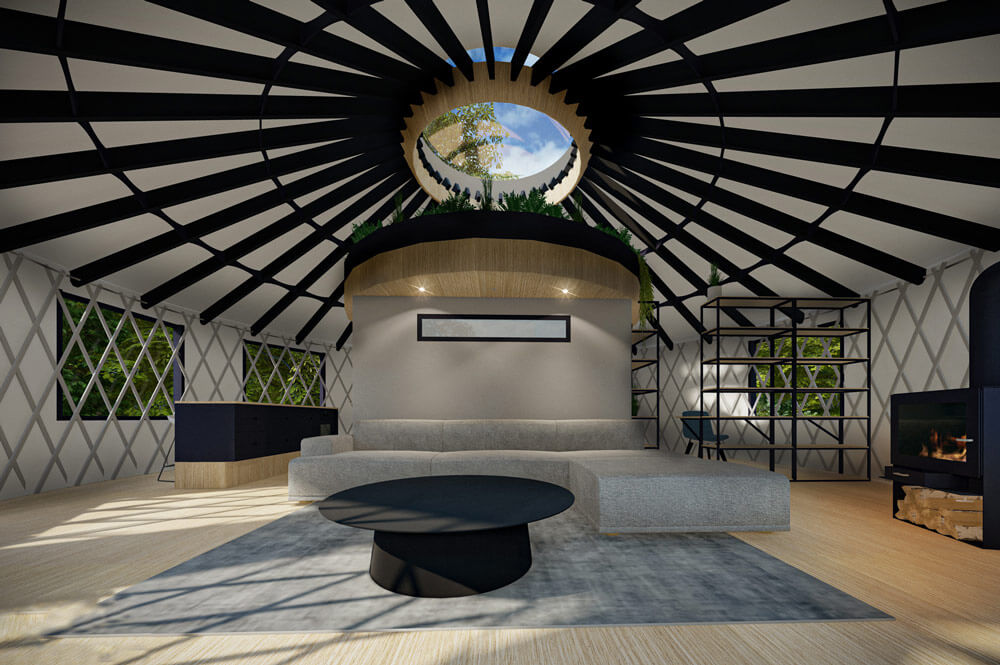This image appears to depict a digitally rendered interior design of a room, possibly a yurt, showcasing a unique and artistic space. The ceiling features a central circular skylight, surrounded by a wooden sunburst design with black metallic spires radiating outward. Below this skylight, a circular podium or stand is positioned in the middle of the room. The room itself is circular, with curved walls adorned with tall windows that offer a view of the trees outside, giving a natural, enclosed feeling.

Covering the windows and walls are intricate gray lattices, adding an interesting, albeit slightly confining, touch to the space. A large, curved gray couch with a chaise lounge on the right creates a cozy seating area in the center of the room, complemented by a black circular coffee table. This arrangement sits on a medium-gray charcoal rug, contrasting with the light pine wooden flooring that surrounds it.

Additionally, to the right side of the room, there is a fireplace or oven neatly stocked with wooden logs below, ready for use. Near the back on the right, storage shelves provide functionality along with aesthetic appeal. This detailed interior combines modern design elements with a harmonious and somewhat rustic vibe, blending form and function in a visually engaging way.